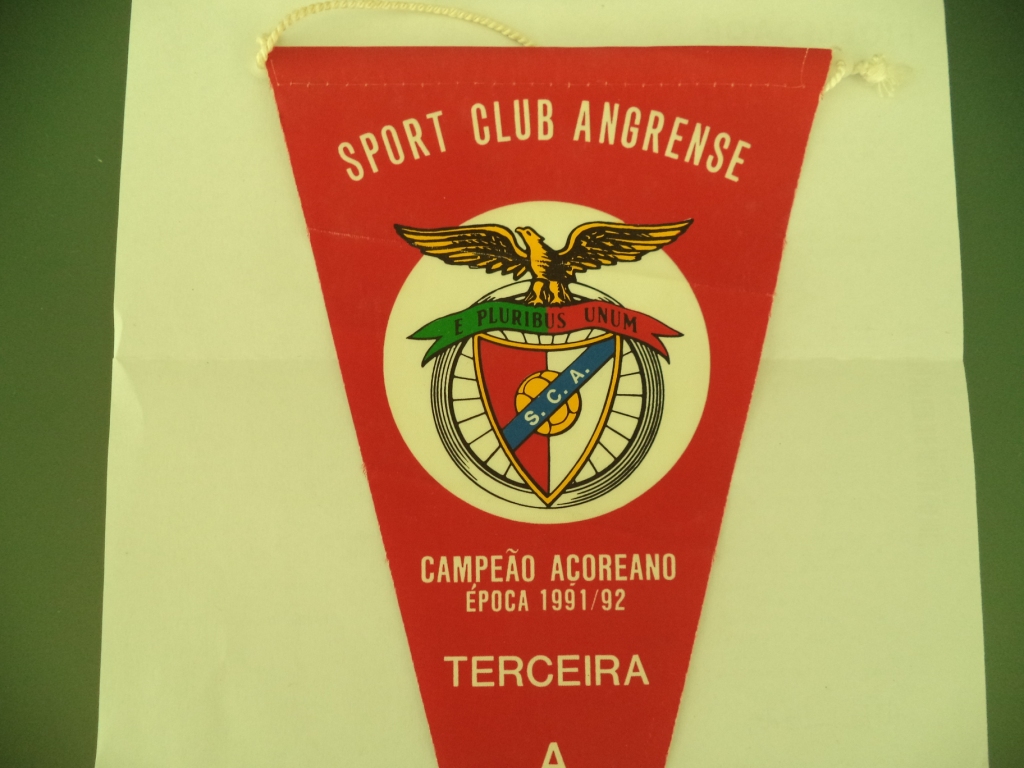This detailed photograph captures a vertically oriented, triangular pennant laid on a folded, whitish-yellow piece of paper, which in turn rests on a green surface. The pennant is a dark red color and features an extensive assortment of text and emblems. At the top, the pennant reads "Sport Club Angrense" in white text. Just below, there is a detailed emblem comprising an eagle perched atop a spiked wheel, with a soccer ball at the center of the wheel. On a blue banner across the soccer ball, the letters "S.C.A." are prominently displayed. Adjacent to the eagle, the text "E Pluribus Unum" is visible. The left edge of the pennant transitions into a green ribbon, while the right edge fades into a red ribbon. Further down, the words "Campião Açoriano" (with tilde over 'a') and "Época 1991/92" are inscribed, followed by the word "Terceira." A whitish-yellow cord at the top of the pennant suggests it can be hung. The entire setup appears to be carefully placed for the photograph, presenting a richly detailed view of this commemorative sports pennant.